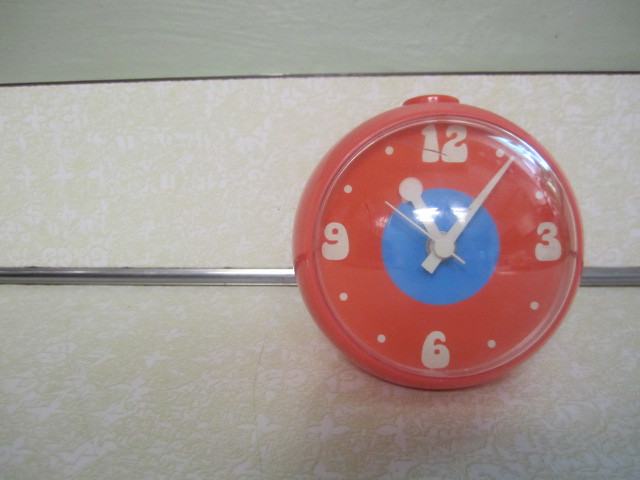The image depicts a uniquely designed clock. The background is divided into three sections: a gray rectangle at the top, a white middle section, and a floral pattern with a silver bar running horizontally through the middle. Positioned on the right side of the image is an eye-catching clock with a red body and face. The clock features the numbers 12, 3, 6, and 9 prominently. The face of the clock is covered with a reflective, bubble-like plastic, adding a distinctive dimension to its appearance. In the center of the clock face, there is a blue dot, and encircling this within the red face is an additional red dot, creating a striking focal point.